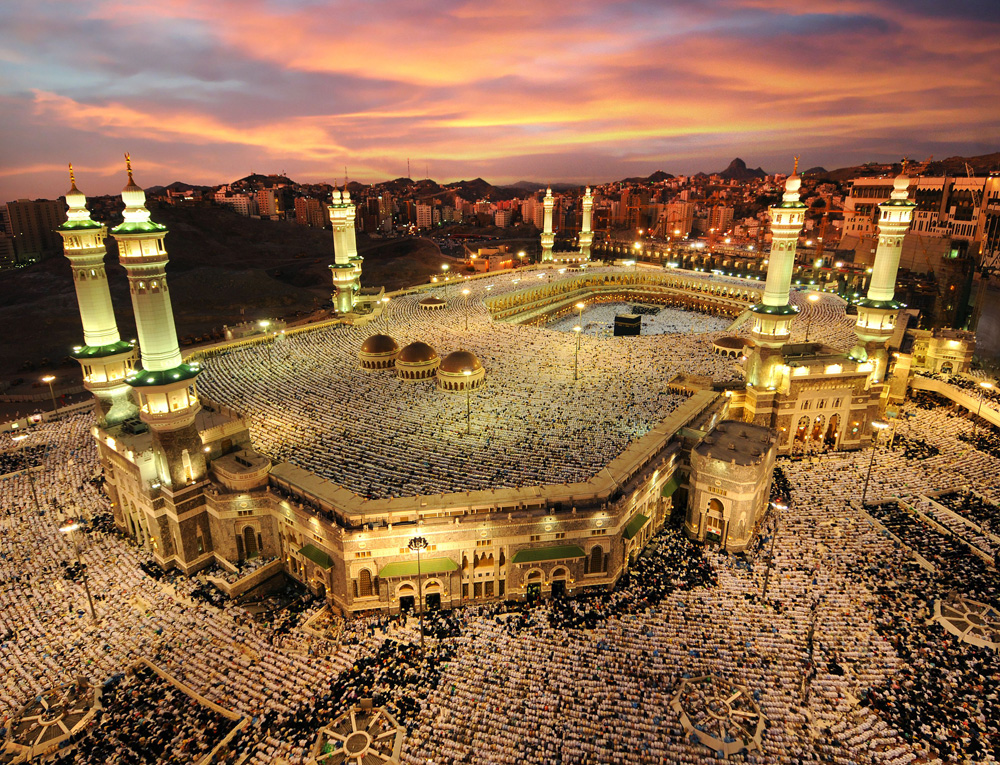This is an aerial photograph, taken at a 45-degree angle, of a modern day castle-like building at dusk, showcasing an intricate, illuminated architectural design. The large, asymmetrical structure in the foreground, which features a geometric pentagon-like front merging into a rectangular back, stands prominently against a vibrant cityscape bathed in the warm hues of a setting sun. The background reveals a sprawling city with buildings that reflect tones of browns and beiges under the orange-pink and yellow-tinged sky, highlighted by streaky clouds with pockets of dark blue.

The main building itself is a striking golden color, adorned with various vibrant illuminations, casting a regal glow. It features tall towers akin to lighthouses or steeples, which are adorned with green and yellow lighting, emphasizing its grandeur. The building appears to be one or possibly two to three stories tall, with turrets and steeples punctuating the skyline. The ground and ceiling surrounding the structure exhibit a tiling pattern in blacks and beiges.

Adding to the unique features, the mansion boasts multiple arched, gold-lined doorways and golden walkways. A cutout in the back middle of the building suggests an open-air area or arena. Gathering crowds and lively ambience hint at an ongoing event, making the sight even more captivating against the ethereal twilight background.